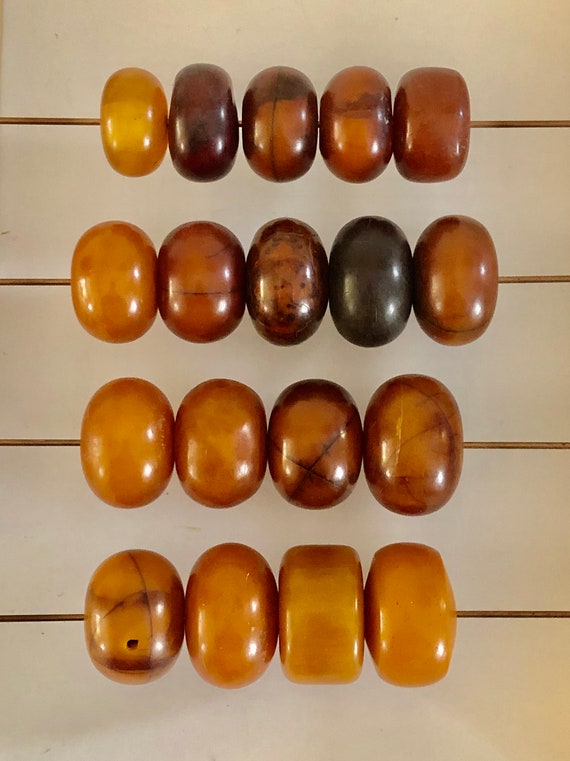The image showcases what appears to be an abacus set against a beige background, featuring four dark wires, potentially coppery black in color, each adorned with beads. The beads vary in size and color, displaying a range of browns, golds, and dark, almost black hues, resembling tortoiseshell patterns. The first and second rows contain five beads each, with the beads in the second row being slightly larger. The third row has four beads that are even bigger and more square-shaped, whereas the fourth row features the largest beads, numbering four and mostly golden-yellow in color. The arrangement suggests a progression from smaller to larger beads across the rows. The diverse shapes and colors of the beads, resembling glass or stone, highlight the functional artistry of this ancient computational device.